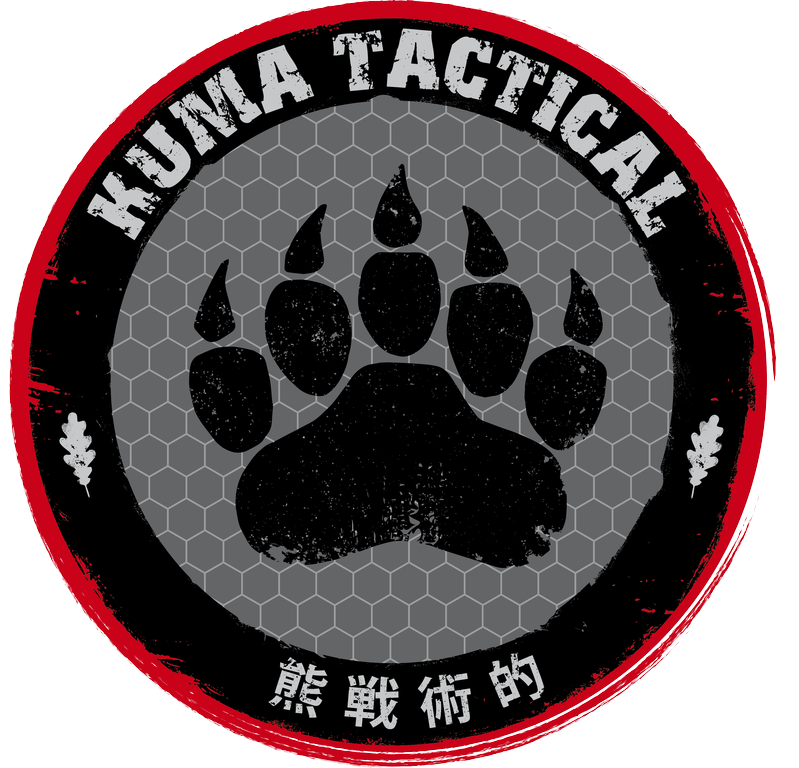This image features a circular logo on a white background, prominently marked by an outer red border with white streaks. Just inside the red perimeter is a black concentric ring, adorned at the top with the text "Kuma Tactical" in white letters. Flanking the left and right sides of this black ring are white illustrations resembling leaves. At the very bottom of the black ring are four characters in an East Asian script, either Japanese or Chinese.

The central part of the logo is a medium gray circle with a light gray, hexagonal pattern reminiscent of a beehive structure. Dominating this central gray area is a large black paw print with visible claws, which appears to be the focal point of the design. The detailed elements, including the red border, the black ring with white text and leaves, the East Asian characters, and the intricately patterned gray background with a prominent paw print, collectively form the distinctive logo of "Kuma Tactical."